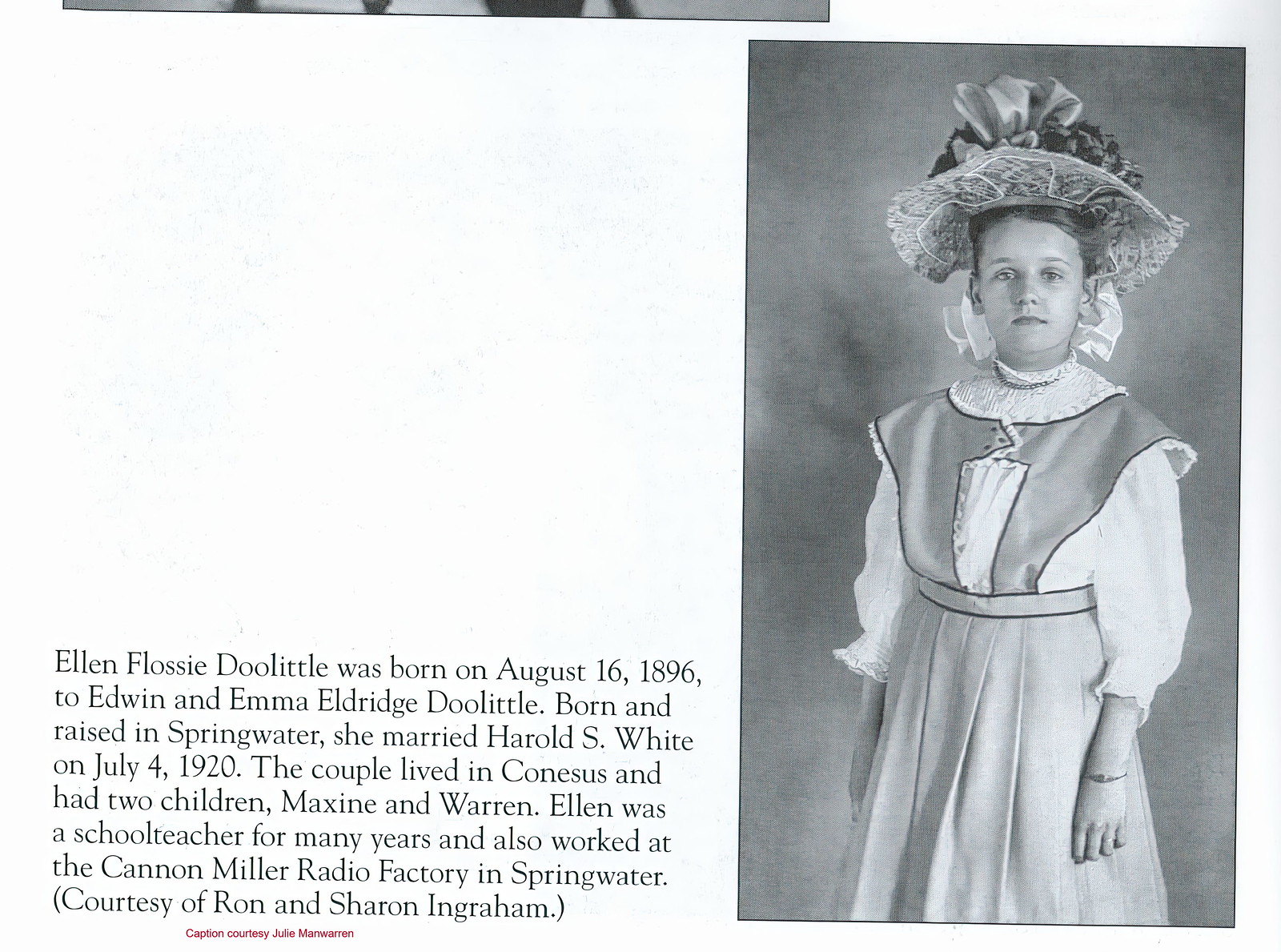The image appears to be a scan from an old newspaper or book page, depicted in black, white, and grayscale. On the right side of the page is a black-and-white photograph of a young girl, Ellen Flossie Doolittle, dressed in a highly elaborate, old-fashioned outfit. She wears an ornate hat adorned with bows and lace, a high-waisted dress featuring a pleated skirt and white sleeves, and a bracelet on one hand. To the left of the image, there's a detailed paragraph of text that provides a biography of Ellen Doolittle. The text reads, "Ellen Flossie Doolittle was born August 16, 1896, to Edwin and Emma Eldridge Doolittle, born and raised in Springwater. She married Harold S. White on July 4, 1920. The couple lived in Conessus and had two children, Maxine and Warren. Ellen was a schoolteacher for many years and also worked at Cannon-Miller Radio Factory in Springwater." An additional note at the very bottom of the image indicates, “Caption, Courtesy, Julie Marwarren” in small red type. The image is shared courtesy of Ron and Sharon Ingraham.